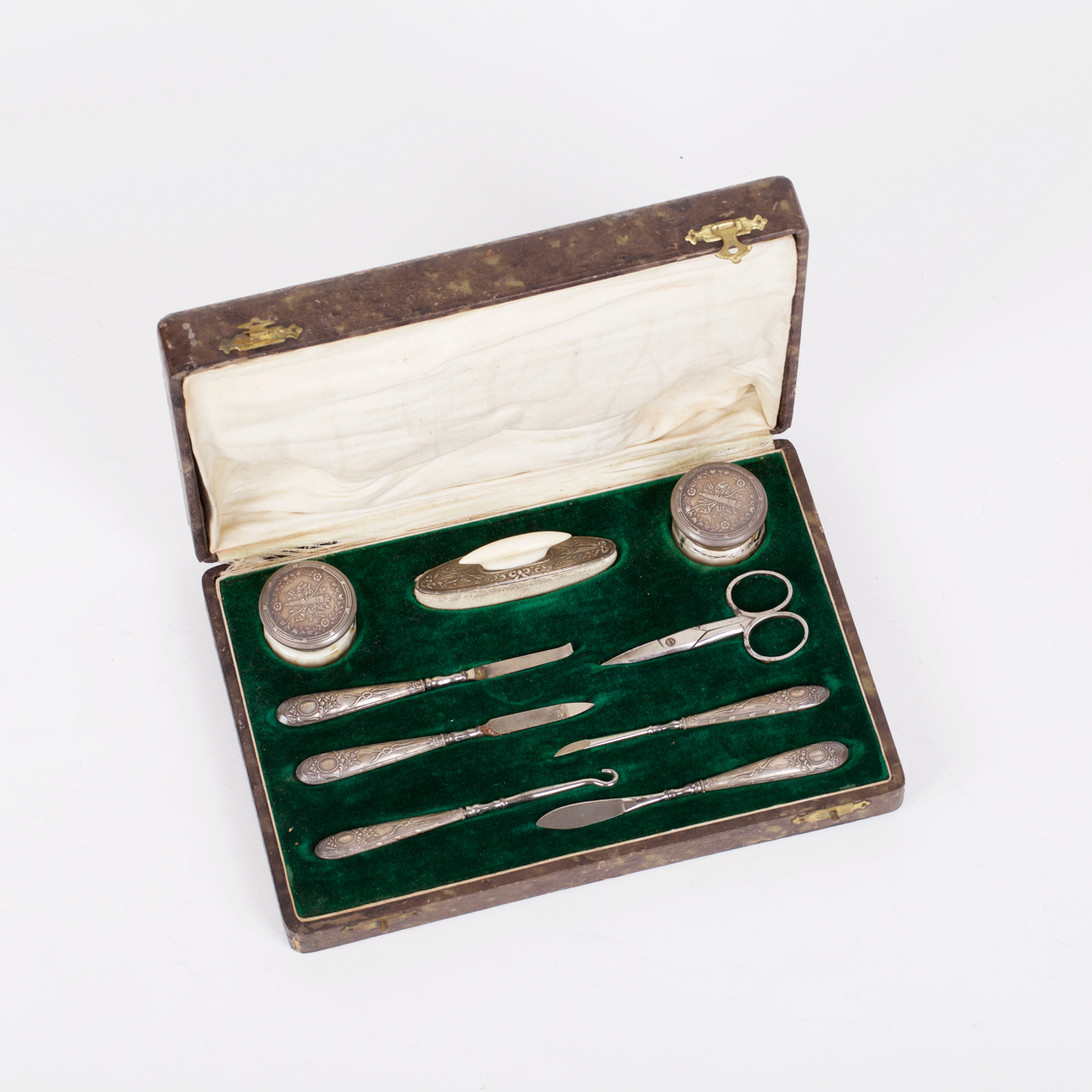This photograph captures a vintage grooming or manicure set housed in an open brown box, reminiscent of a small chest or storage container. The box, measuring approximately the size of a shoebox but only about two to three inches in height, is placed against an off-white to light gray background. The image is taken from above, allowing a clear view of the contents and the intricate details of the set.

Inside the box, a weathered white cloth lines the top lid, exhibiting yellowish spots. The outer casing appears to be made of a brown material with varying shades, giving it a wooden texture with hints of yellow. The base of the interior is lined with green velvet, in which various grooming tools are meticulously arranged.

Among the tools, there is a pair of small silver scissors with large finger openings and tiny blades. Alongside the scissors are several flat devices, each boasting an ornate handle with distinctive functions; one appears to be a nail file, another has a pointed end, possibly for cleaning nails, while another features a small hook. Additionally, two round metal jars occupy the top corners of the box. The items, mostly silver with hints of bronze, suggest age and classical design.

The box is secured with two golden metal latches at the top, complementing the gold hinges at the back. This intricately crafted set, combining practicality with antique charm, reflects its historical essence and delicate craftsmanship.